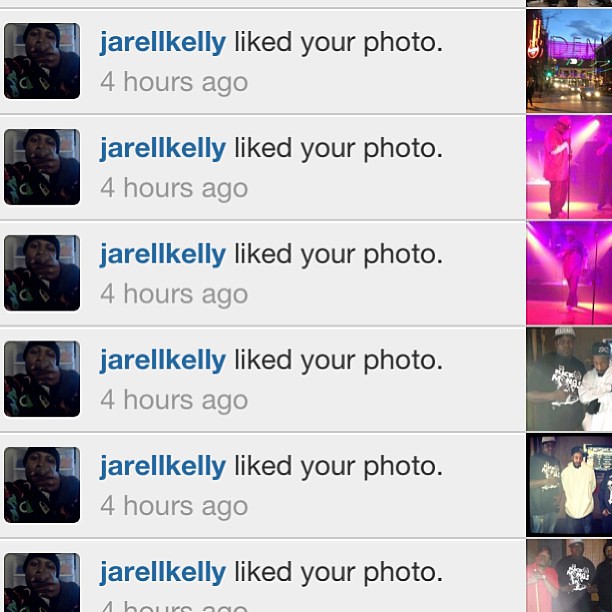This image is a screenshot from someone's Instagram notifications feed, showcasing a series of six notifications from a user named Jarell Kelly, who liked multiple photos four hours ago. On the left side, Jarell Kelly’s profile picture appears repeatedly; he is a young African-American male, likely in his early 20s, posing with his fingers pointed forward in a gun shape. The right side displays the photos he liked: starting from top to bottom, there's a nighttime street view with cars, two images of a singer performing under purple stage lights, and then three group pictures. Notably, the group photos show African-American individuals, with one person in a black and white shirt possibly being the same singer featured in the concert images. The screenshot itself appears to be from an older version of Instagram.